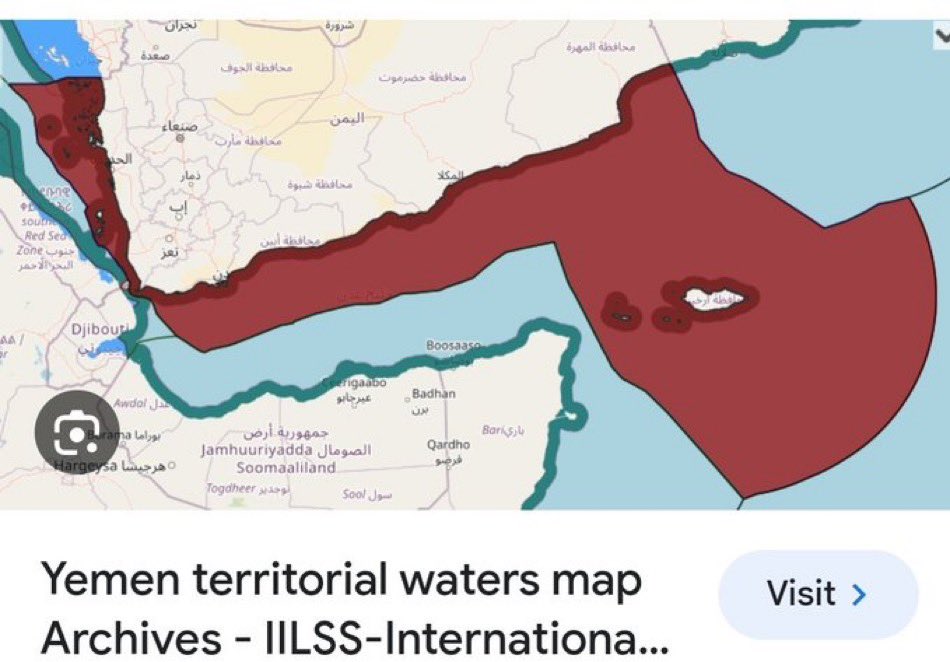The image features a detailed map predominantly colored in shades of blue, red, burgundy, and gray, delineating the territorial waters and landmasses of Yemen. The land areas on the map are outlined in dark green and are shown in an off-white color. Bodies of water are depicted in various shades of blue, with a prominent deep red, almost burgundy, area positioned between two main landmasses and extending downwards to the right. On the map, names of provinces and cities are written in an Arabic script; a few names are discernible, such as Badam, Quadho, and Djibouti, hinting at a connection to the Red Sea Zone. A dark gray circular icon resembling a camera, indicating a Google Image search result, is located in the bottom left corner. Directly above this icon, black text reads “Yemen Territorial Waters Map Archives IILSS International,” followed by an ellipsis. Nearby, a "Visit" button with a directional arrow suggests navigation options.